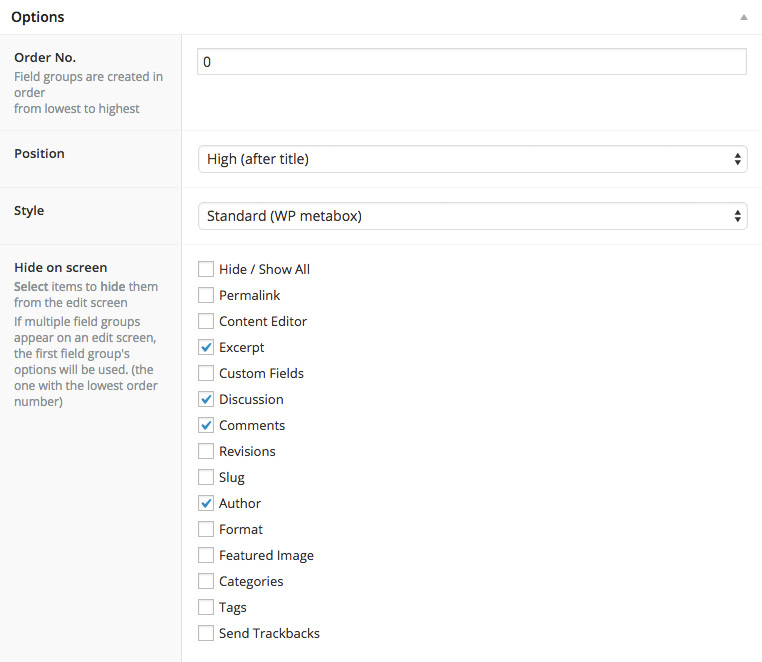The image displays a user interface screen titled "Options" in bold black text at the top. Below the title, on the left side, there is a vertical menu bar featuring several categories: "Order Number," "Position," "Style," and "Height on Screen." 

On the right side, set against a white background, each category has corresponding selection fields:

1. "Order Number" features a number input field.
2. "Position" is represented by a drop-down box, with the current selection set to "High, After Title."
3. "Style" also has a drop-down box, currently showing "Standard, WP Meta Box."
4. "Height on Screen" provides approximately 15 different checkboxes, of which four—namely "Excerpt," "Discussion," "Comments," and "Author"—are checked. 

This detailed depiction highlights the configuration options for a specific system or application interface, though the exact purpose of the screen remains unspecified.